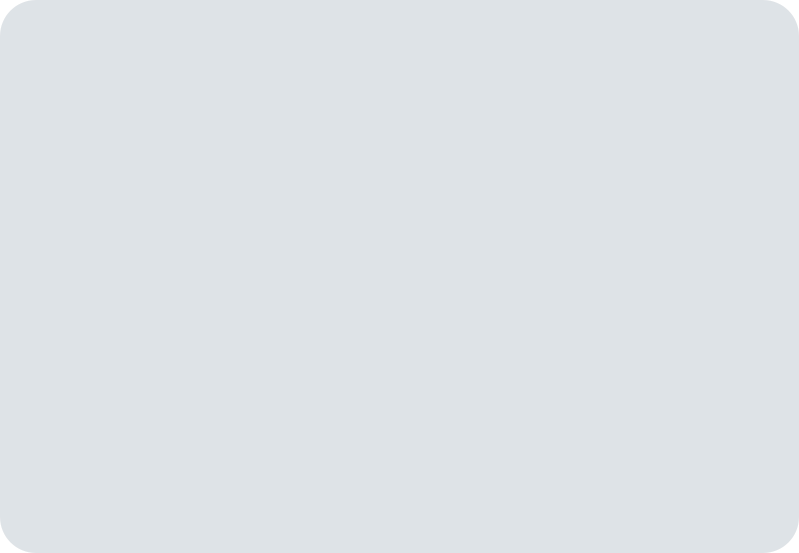A solid square of a bluish-gray color dominates the image. The square has smooth, rounded edges on each corner, and there is absolutely nothing else within the frame. There are no details, textures, or additional elements to distract from the simplicity of the square's design.